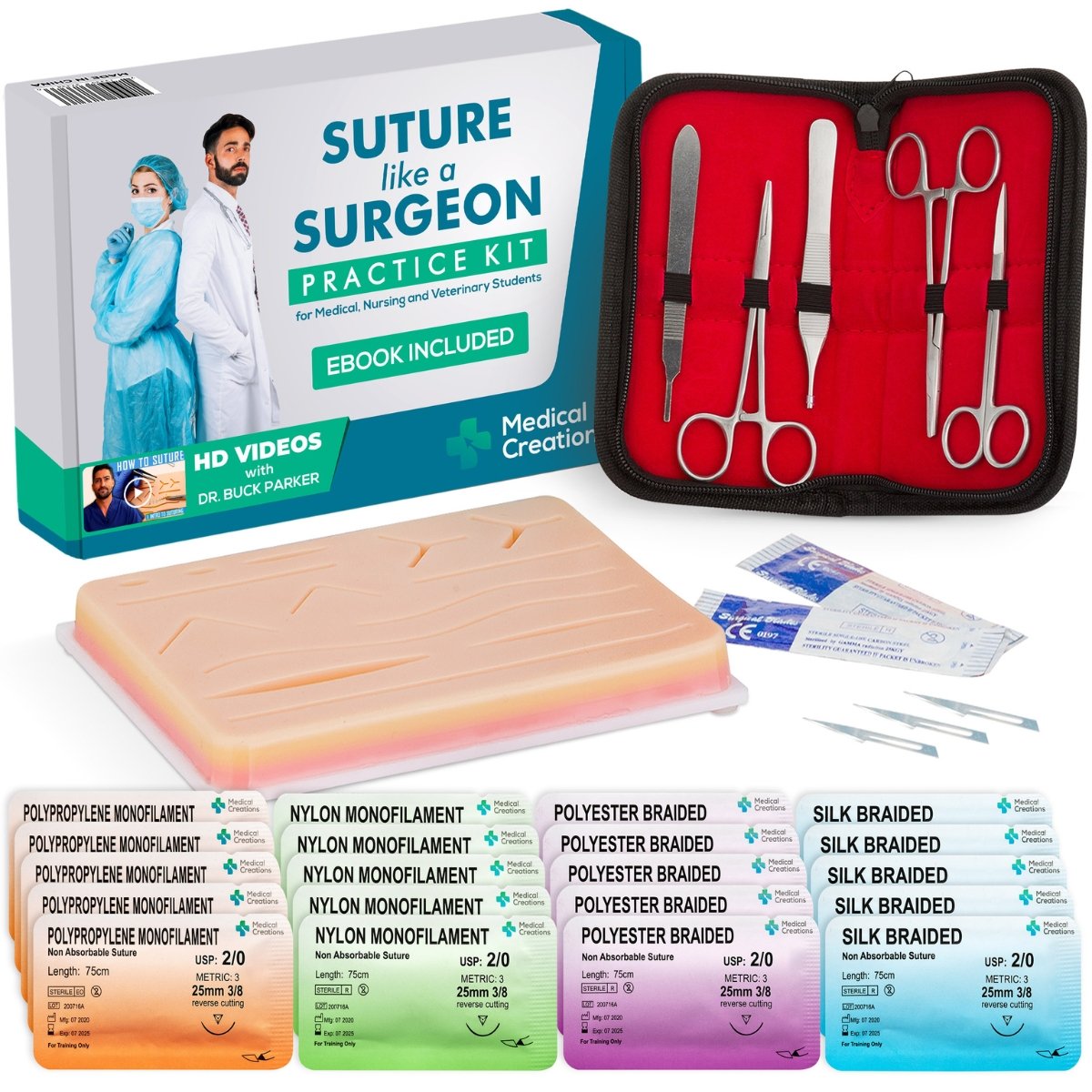The image displays an expansive suture practice kit designed for medical, nursing, and veterinary students. Dominating the top section is a gray and blue box featuring the kit, prominently titled "Suture Like a Surgeon" in vibrant blue lettering. The cover showcases a woman in scrubs with a face mask and a man in a white coat, alongside the text highlighting the inclusion of an e-book and HD videos by Dr. Buck Parker. The bottom right corner of the box is branded with "Medical Creations" accompanied by a symbol.

Adjacent to the box on the right, there is an open black bag containing five instruments: three types of scissors and two tools resembling files. An upside-down plastic tray is visible in front of the bag, likely for practice suturing. To its right, there's a cluster of small plastic packets, seemingly three brushes.

Lower in the image, there are four rows of small rectangular packets, each row containing five packages. These include an orange packet labeled with "polypropylene monofilament" (partially visible), a green packet for "nylon monofilament," five purple packets with "polyester braided," and five blue packets with "silk braided." Additionally, the image showcases a silicone suture pad with various incisions for practical training.